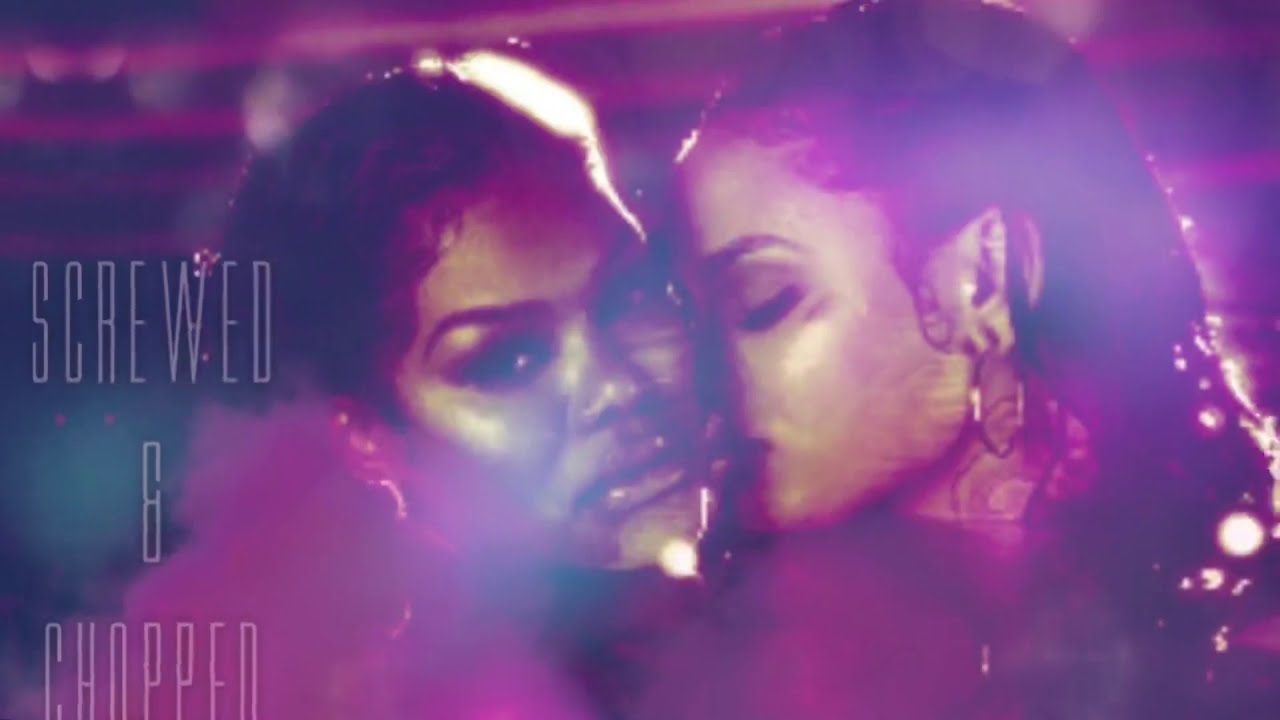The image displays two African-American women under a light purple and dark navy blue background, both with shiny, light-reflective hair. They are depicted in a color scheme dominated by pinks and purples, with both women wearing earrings. One woman is looking directly at the camera, while the other is leaning in romantically towards her, almost as if she's smelling her. On the far left, there is stretched, capitalized text in gray that reads "SCREWED & CHOPPED." The atmosphere is enhanced by what appears to be purple smoke, adding a dreamy, ethereal quality to the scene.